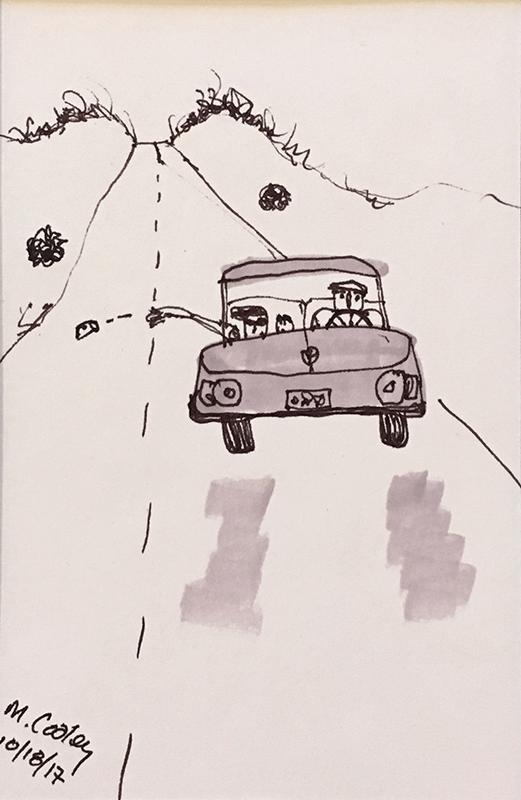This is a detailed hand-drawn picture on cream-colored, vertically aligned rectangular paper. At the bottom left corner, it is signed "M. Cooley" with the date "10/18/17." The drawing features a gray-shaded car with black outlines, driving towards the viewer on a two-lane road. The road is depicted with black dashed lines in the center and solid black lines on each side. In the car, there are three figures: an adult male driver with a hat, an adult male passenger with black hair sticking out, throwing a can out of the window, and a small child visible only by the head, seated in the back. The car has small wheels and features like headlights and a license plate are drawn in. Surrounding the road, there are squiggly lines and bushes suggesting hills and grass. The paper shows a slight brown stain at the top edge, adding to the impression of age or use. This drawing, likely created by a child, portrays a simplistic yet detailed scene of a family drive.